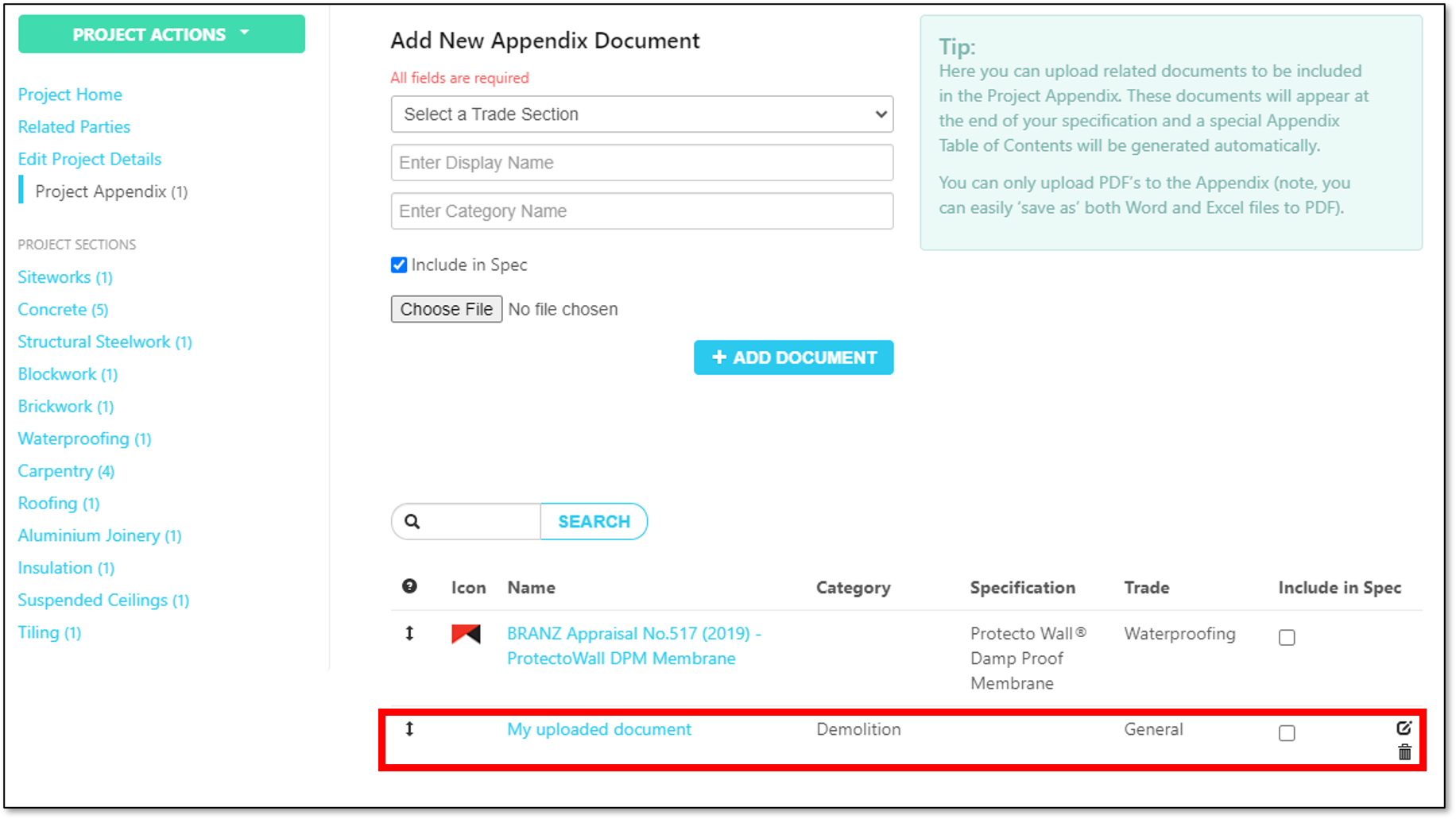The web page features a predominantly white background, with various interactive elements for managing project documents. In the lower right corner, a red-outlined square highlights a specific area of interest: within this square is an uploaded document titled "Demolition General." Adjacent to this document's title is a checkbox, and to the right of this checkbox are two icons—a trash can symbol for deletion and an edit symbol.

In the top left corner of the page, there's a button labeled "Project Actions," which serves as a dropdown menu for additional options. Next to this is another prompt, "Add New Appendix Document," which requires the user to complete several mandatory fields, including "Select a Trade Section" (a dropdown menu), "Enter Display Name," and "Enter Category Name."

Below these input fields, there's a checked blue checkbox labeled "Include in Spec." The section continues with a "Choose File" button, allowing users to upload a file from their computer.

The lower portion of the control panel lists several sections with the headers: Icon, Name, Category, Specification, Trade, and Include in Spec.

Overall, the page is designed for document management within a project, offering various features to upload, categorize, and edit files.